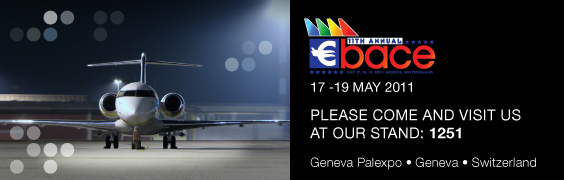The image is a horizontally aligned advertisement, resembling a small rectangular ticket, approximately 6 centimeters by 14 centimeters. It is split into two equal halves. On the left side, there's a high-resolution image, potentially a photograph or a very detailed digital rendering, of a jetliner facing directly towards the viewer. The airplane's engines are visible at the rear, with a prominent cockpit featuring a long black horizontal window. The aircraft is illuminated by a spotlight, casting a pool of light and creating a dramatic effect. The background of this segment is mostly black at the upper part, transitioning to gray at the bottom third, with additional elements such as storage sheds with orange fronts, and scattered blue, light gray, and dark gray circles.

On the right side, the background is black with a gradient pattern of rainbow-colored triangles, shifting from blue to red, located at the top. Below these triangles are two horizontal blue dotted lines with a white Euro sign nestled between them on a blue square background, and text indicating "15th Annual" on a small white banner. The prominent red lowercase letters "bace" stand out, with the preceding "E" forming "E-bace." Below that, the date "17 to 19 May 2011" is displayed in uppercase letters. Further down is an invitation in larger white text: "Please come and visit us at our stand, call in 1-2-5-1." The bottom section reads in mixed case: "Geneva Palexpo, Geneva, Switzerland," noting that the event is to be held at a modern venue which suggests it is a contemporary event within the last decade.